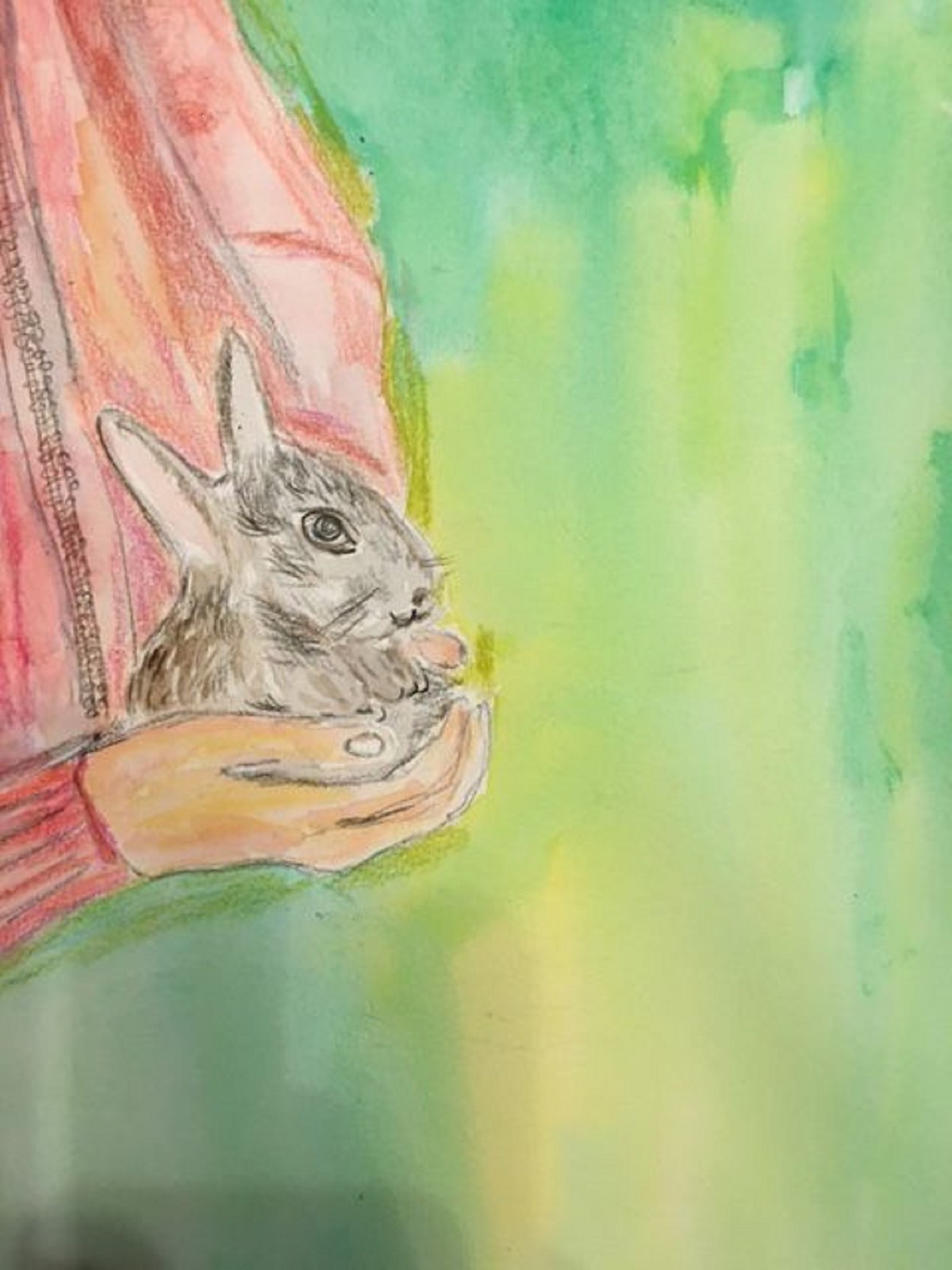The image is a detailed and striking watercolor and color pencil artwork. The left side features a woman wearing a red-pink sweater, which exhibits varying shades of red, characteristic of watercolor painting. Her left hand, watercolor-painted in a peach-beige tone, is depicted holding a small, gray bunny. The bunny, rendered in color pencil, has big ears and a content expression on its face, with one eye visible. The background shifts from various shades of grass green to a lighter lime green, all painted with watercolors, creating a serene and harmonious backdrop. There is no text in the image, and the overall composition, from the detailed textures of the sweater to the soft hues of the background, enhances the tender moment captured between the woman and the bunny.